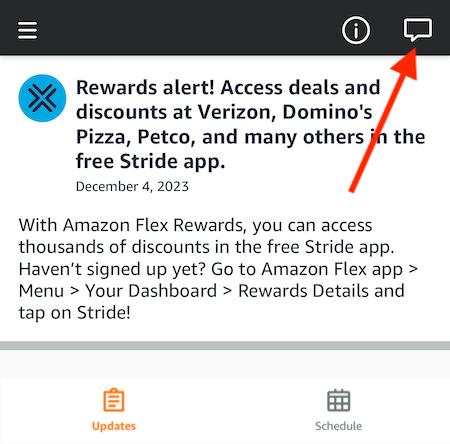**Rewards Alert!** Access deals and discounts at Verizon, Domino's Pizza, Petco, and many others in the free Stride app.

*December 4, 2023*

At the top of the image, a black bar serves as the header. On the left, three white lines signal a drop-down menu, while on the right, a white circle with a lowercase "i" offers additional information upon clicking. Adjacent to the "i" icon, a white comment blurb icon is highlighted by a red arrow originating from a grey box of text.

The grey text reads: "With Amazon Flex Rewards, you can access thousands of discounts in the free Stride app. Haven't signed up yet? Go to Amazon Flex App, navigate to your dashboard, rewards details, and tap on Stride!" 

Immediately below the header, there is a strip of light grey, followed by a larger off-white section. In the bottom left of this section, an orange clipboard icon with lines resembling writing indicates "Updates." On the right, a clip art icon of a calendar labeled "Schedule" is visible.

On the far left of the header, a blue circular icon with a black-bordered "X" marks the close button.